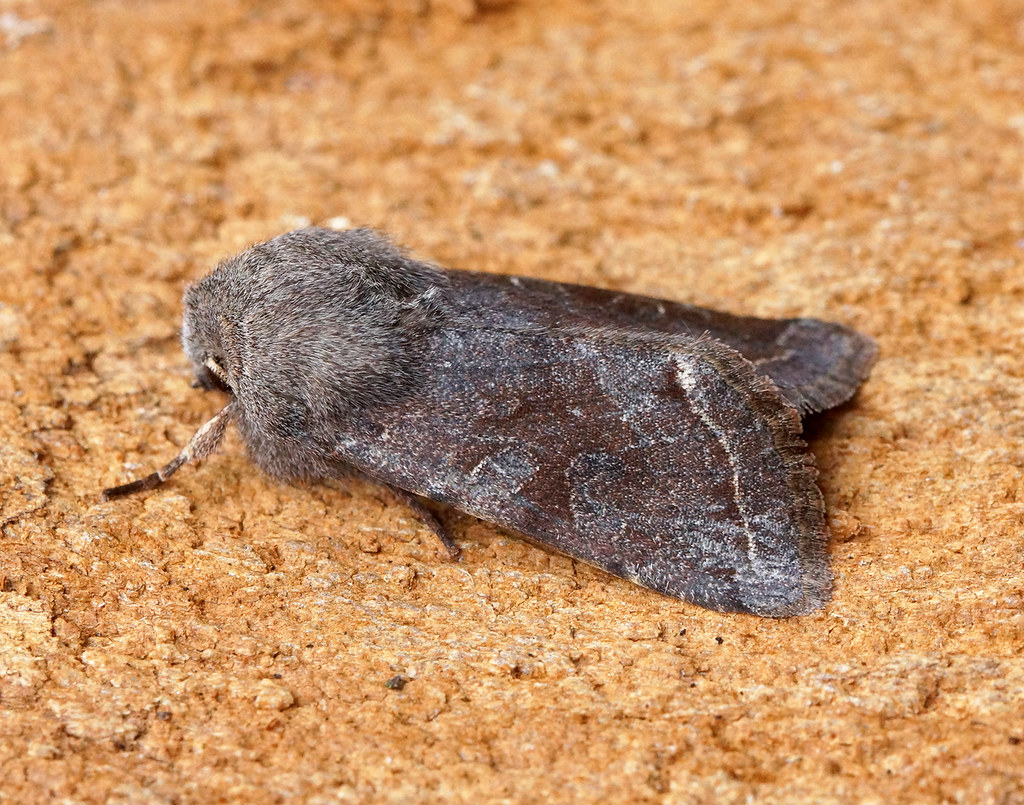This is an extreme close-up image of a moth perched on a porous, rock-like surface of light brownish color with darker bits and lighter streaks. The moth is centered in the photograph, displaying its closed wings tucked near its back and its head tilted up and to the left. The moth's body and wings are predominantly dark brownish-gray, with the wing centers being a darker brown and the tips displaying frosted gray hues with ridges of dark brown similar to its abdomen. Fine, light grayish hairs envelop its head, adding texture to its appearance. Two legs are visible protruding from beneath its body and wings—one leg appears white at the top, transitioning to brown towards the foot, while the other leg is mostly brown and thin. The moth's overall coloration is a mix of dark tones with lighter grayish streaks and splotches, giving it a subtly mottled look.